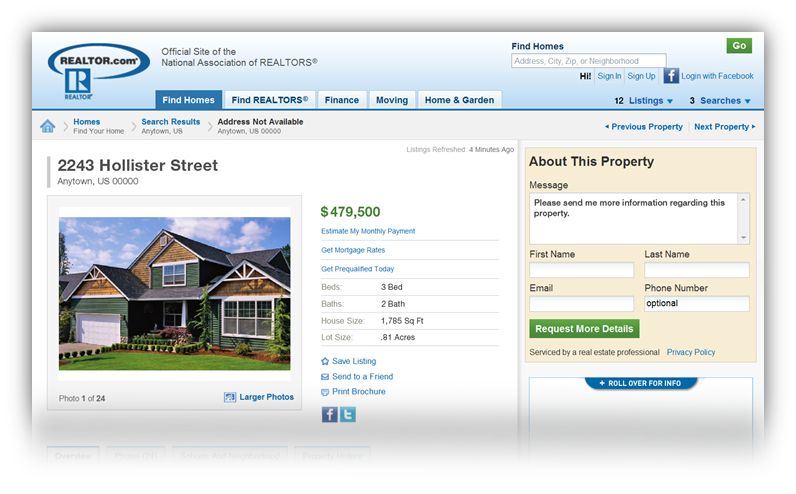Screenshot of the Realtor.com homepage displaying the header with the Realtor.com logo and the tagline "Official Site of the National Association of Realtors." The navigation menu features tabs labeled "Find Homes," "Find Realtors," "Finance," "Moving," "Oven," and "Garden," with the "Find Homes" tab highlighted in blue. The main content showcases a large, modern house with the address "2243 Hollister Street, Anytown, USA, 00000," listed for $479,000. The sidebar includes a section titled "About This Property" and a form to send a message to the Realtor.